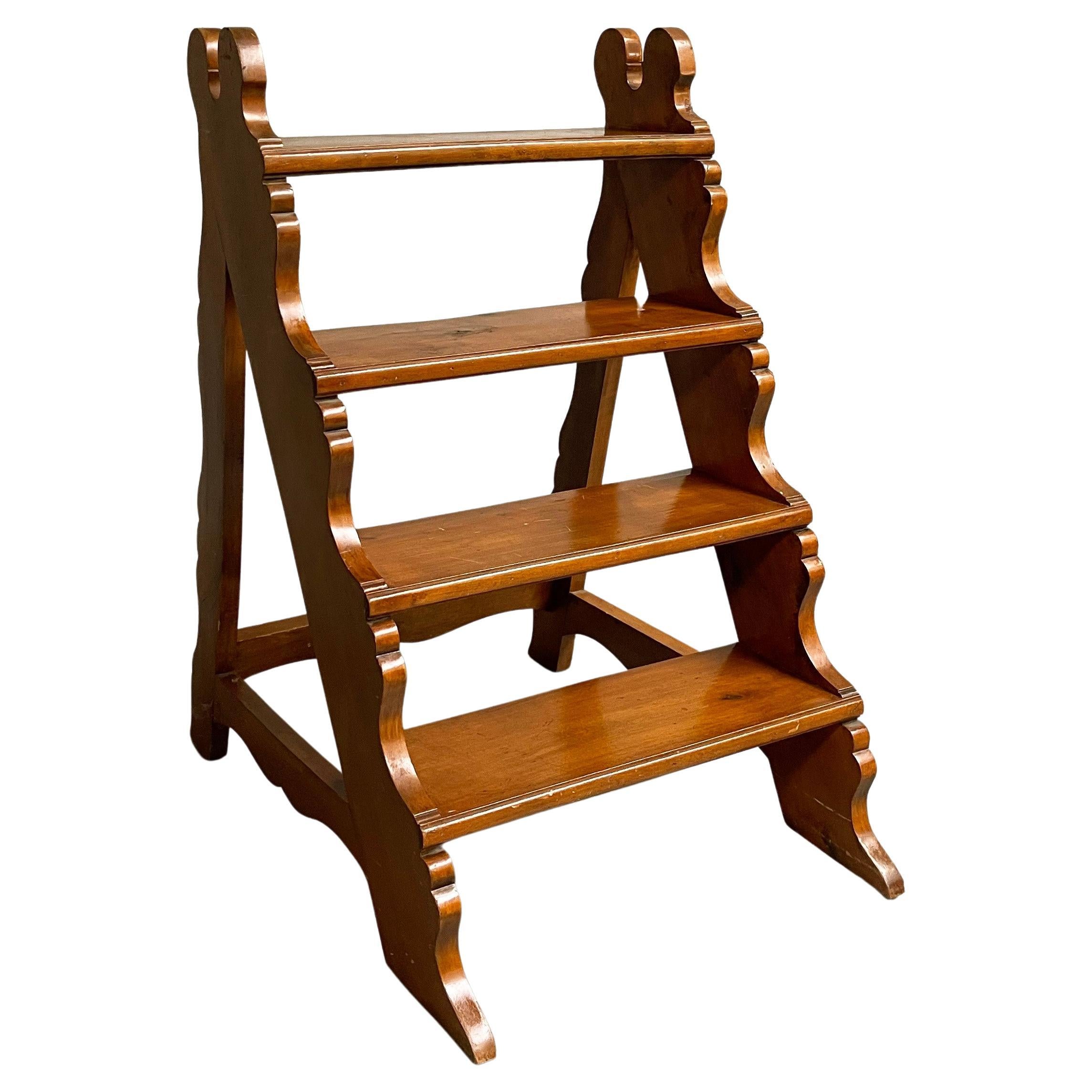This image features a vintage-style wooden stepladder with four steps, characterized by a medium to dark brown stain that highlights its natural wooden markings, including some knot spots on the lower steps. The stepladder is adorned with decorative, almost swirly, carvings along the edges, giving it a charming, handcrafted appearance. It stands on a clean white background, enhancing its visibility and emphasizing its intricate details. The structure includes supportive beams bridged along the sides and the back, and it is designed to resemble a small, stationary step stool, possibly for reaching higher cabinets or as a decorative plant stand. The top step, shaped almost like two little ears, is somewhat obscured due to the angle of the photograph, while the lower three steps are more clearly visible.